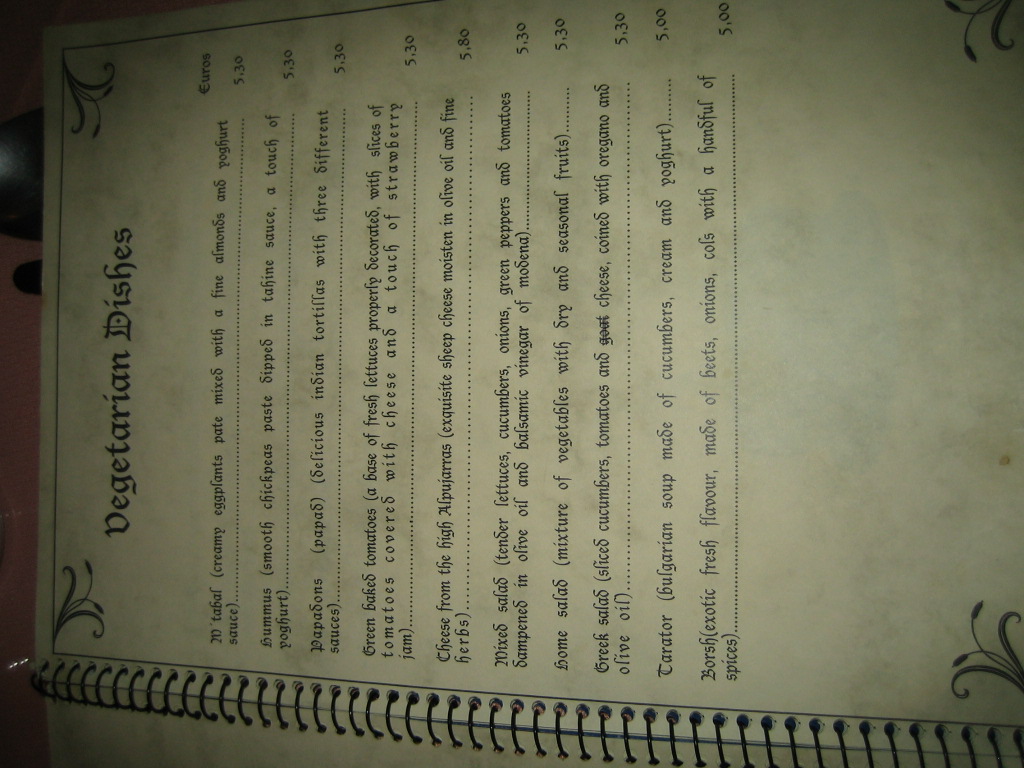This photograph captures a detailed page from a spiral-bound cookbook or menu, showcasing an array of enticing Vegetarian Dishes. The page, printed on white paper with black text, features its title elegantly scripted at the top. 

The dish names, listed from top to bottom, include:

- **Falafel** 
- **Hummus**
- **Papadones**
- **Green Baked Tomatoes**
- **Cheese from the High**
- **Aloo Haras**
- **Mixed Salad**
- **Home Salad**
- **Greek Salad**
- **Taratar**
- **Borscht**

Each dish is accompanied by a small, descriptive script providing a brief explanation or ingredients of the dish. Decorative flowers embellish the borders of the page, adding a touch of charm and visual interest. This image encapsulates the essence of a well-curated vegetarian menu or section from a cookbook.